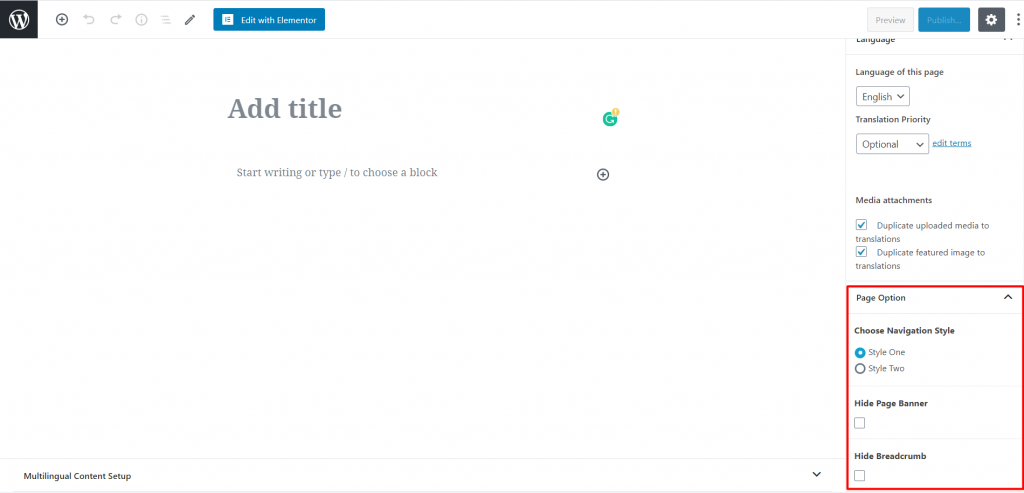A screenshot captures the interface of a dialogue from an unidentified application. Dominating the top left is a logo marked with a "W," potentially representing Wikipedia. Adjacent to this logo are several icons: a plus sign, a left curved arrow, a right curved arrow, an information icon, a three-line indentation (likely representing a menu), and a pencil poised for editing. A notable feature is a prominent blue button labeled "Edit with Elementor."

On the upper right side, additional controls are visible, including a "Preview" option, another blue button with unclear text, a gear icon inside a gray box, and a vertical ellipsis indicating more menu options.

Beneath this menu bar, the main content area is predominantly white, displaying prompts such as "Add title" and "Start writing or type to choose a block." To the right of this main content section is a menu interface. The first item is a language selector labeled "Language of this page," currently set to English. Below it, a selection box for "Translation priority" is set to "Optional."

Following this are options for media attachments, featuring a couple of checkboxes. Encased in a red outline box at the bottom are various page options: "Choose navigation style" with selectable styles labeled "Style 1" and "Style 2," as well as toggle options for "Hide page banner" and "Hide breadcrumb."